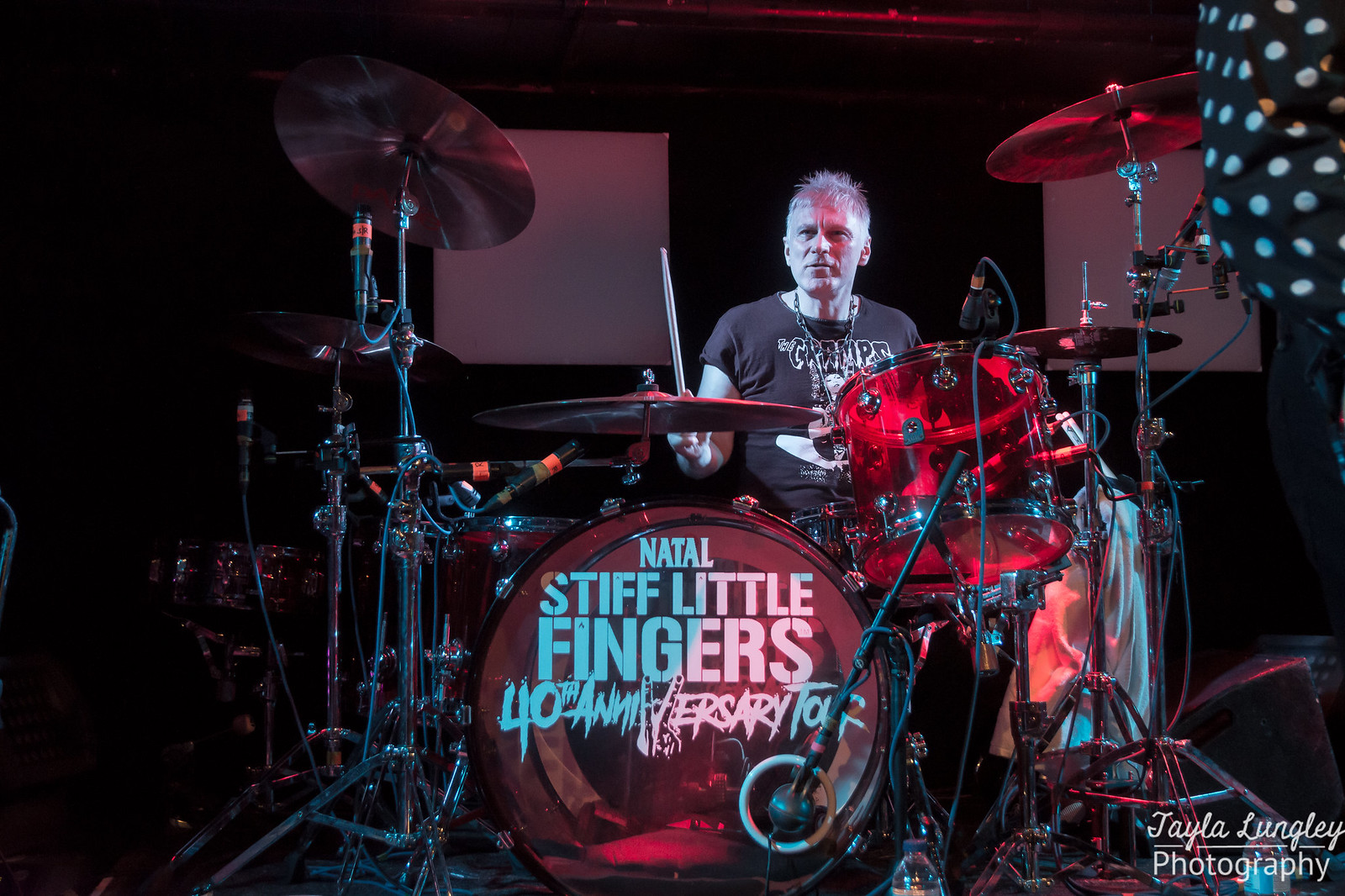This photograph captures a drummer seated behind an elaborate drum kit. The drummer, who has short gray hair and is smiling, is wearing a black t-shirt with the word "Gramps" printed on the front. Around his neck is a lanyard. He holds a drumstick in his right hand. The drum kit is an extensive setup featuring transparent drums with a red theme, various cymbals, and a bass drum, among other paraphernalia, including wiring and speakers. The backdrop is dark, with two screens faintly visible. Prominently displayed on the front of a large red drum are the words "Natal Stifling Fingers 40th Anniversary," indicating a connection to the band Stiff Little Fingers. In the lower right corner, the text "Taylor Langley Photography" credits the photographer.